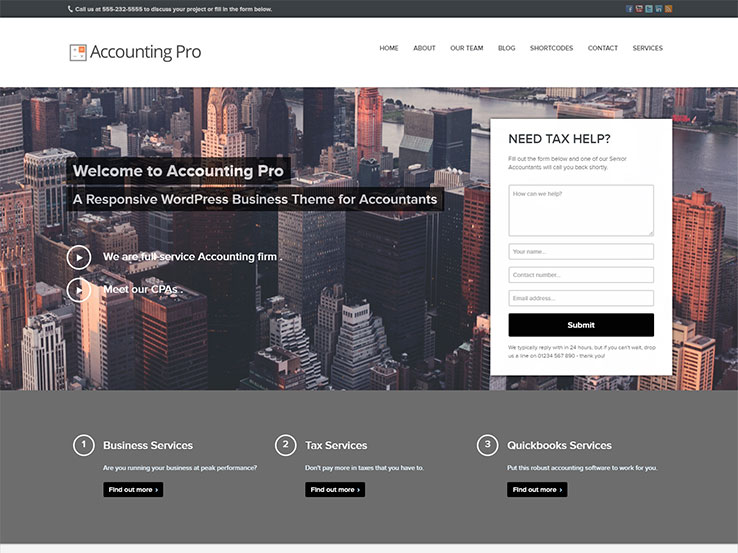This is a screenshot of the website Accounting Pro.

At the top of the screenshot, there is a black banner featuring a phone icon and a call-to-action in white letters that reads, "Call us at 555-222-0555 to discuss your project or fill in the form below."

Beneath the banner, the website's logo and name, "Accounting Pro," are prominently displayed in black letters against a white background. To the right, there is a horizontal navigation menu with several tabs labeled: Home, About, Our Team, Blog, Short Codes, Contact, and Services.

The main content area showcases a captivating image of a city's skyline taken from an elevated perspective, giving a bird's-eye view of the urban landscape. Overlaying this image is a welcoming message in bold white letters that reads, "Welcome to Accounting Pro. A responsive WordPress business theme for accountants."

On the right-hand side of the screen, within a white rectangular box, there is a prompt that reads, "Need tax help?" followed by a form for visitors to fill out and a prominent "Submit" button.

At the bottom of the screenshot, an additional navigation menu is visible, including tabs for Business Services, Tax Services, and QuickBooks Services.